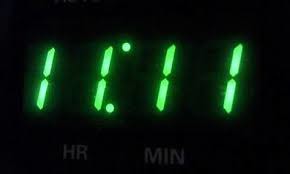This is a detailed photograph of a digital clock, taken up close so that only the display is visible. The clock has a pitch-black face with bright green numbers prominently showing the time 11:11. Each digit is formed by two parallel green dashes, creating a distinct design with a black line running through their centers. The colon separating the hours from the minutes features two dots: the top dot is slightly higher than the digits, while the bottom dot is lower. At the very bottom of the display, in subtle gray lettering, are the abbreviations "HR" for hours, located beneath the first pair of ones, and "MIN" for minutes, positioned beneath the second pair. The stark contrast between the vivid green digits and the jet-black background draws immediate attention to the display, celebrating the symmetrical moment of 11:11.